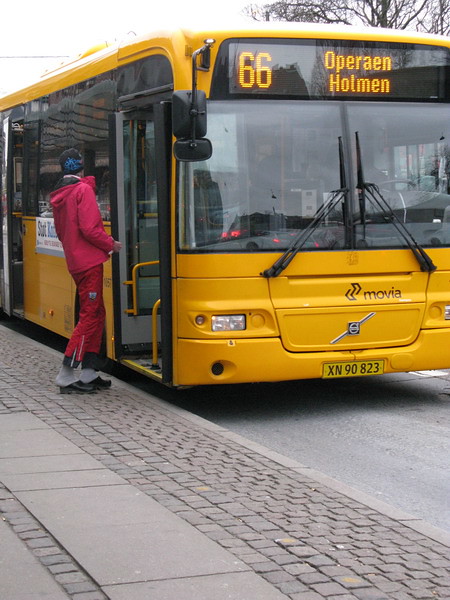In this vibrant urban scene, a bright yellow, modern city bus occupies the top two-thirds of the image, with the remaining portion depicting a sidewalk featuring two dark gray strips of brick amidst an otherwise gray expanse. The bus displays '66' in bold yellow type on a black digital screen at the front, followed by 'Operion Holman' across two lines, although the exact wording might vary slightly. The front window of the bus reflects light, obscuring the driver from view. Below this window, a logo that resembles directional arrows and the name 'Movia' are visible, with an additional indiscernible silver logo beneath it. The bus has black windows along the upper half, adorned with a white banner containing blue text that is difficult to read. 

On the sidewalk, a tall, slender figure dressed in a striking red ensemble, consisting of a parka and track pants, stands poised to board. They wear gray socks and black clogs that appear too small, with their heels spilling out the back. The bus door is open, welcoming the passenger who is possibly engaging with the driver as they prepare to embark.